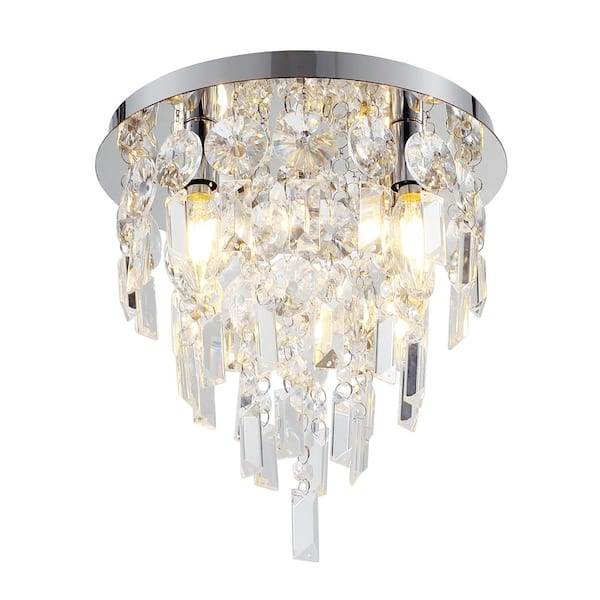This image features a chandelier suspended against a stark white background, making it the sole focus of the photograph. The chandelier's main structure is a glossy, cylindrical silver base that attaches to the ceiling. This base is reflective and shiny, enhancing the visual appeal. Hanging down from this base are numerous glass and crystal elements, including rows of smaller, round diamond-like jewels and rectangular glass pieces. These components catch and reflect light, creating an array of sparkling reflections.

There are two light bulbs visible, positioned symmetrically to the right and left of the chandelier's center axis. The entire fixture forms an inverted triangular or cone shape, tapering to a point at the bottom where a larger rectangular piece of glass is noticeable. Colors in the chandelier include various shades of yellow, off-white, silver, and gray, with slight hints of black, contributing to its shimmering and glittering effect.

The overall image does not contain any text or additional subjects, ensuring the chandelier remains the focal point. The light is bright and reflective, but the context of whether the image was taken indoors or outdoors, or during the day or night, remains undetermined, possibly lending the image a somewhat surreal or computer-generated quality.